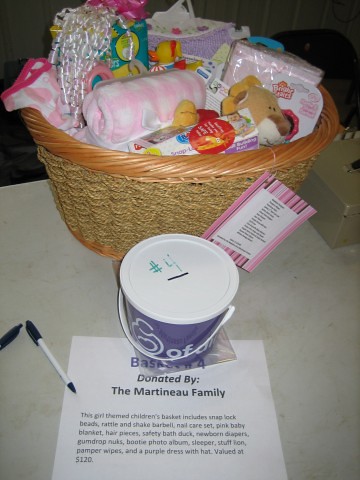The image features a beautifully assembled baby gift basket, prominently donated by the Martineau family for a charitable auction aimed at supporting new mothers. The basket, themed for a baby girl, is brimming with thoughtful items, showcasing a pink baby blanket, a safety bath duck, a snug onesie, and wipes among various other baby essentials. Additional highlights include snap lock beads, a rattle and shake barbell, a nail care set, delicate hair pieces, a stuffed lion, newborn diapers, gumdrop nuts, and a cozy sleeper. The gift set also features a charming purple dress with matching hat, a photo album, and pamper wipes. Accompanying the basket is a small purple donation bucket with a coin slot, emblazoned with March of Dimes branding, indicating its role in the fundraising efforts. A neatly placed sheet of paper beneath the bucket identifies the basket as number four and lists a detailed inventory of the contents, valuing the basket at $120. This well-curated basket, prepared for an auction, reflects the generosity of the Martineau family and the community's support for the cause.